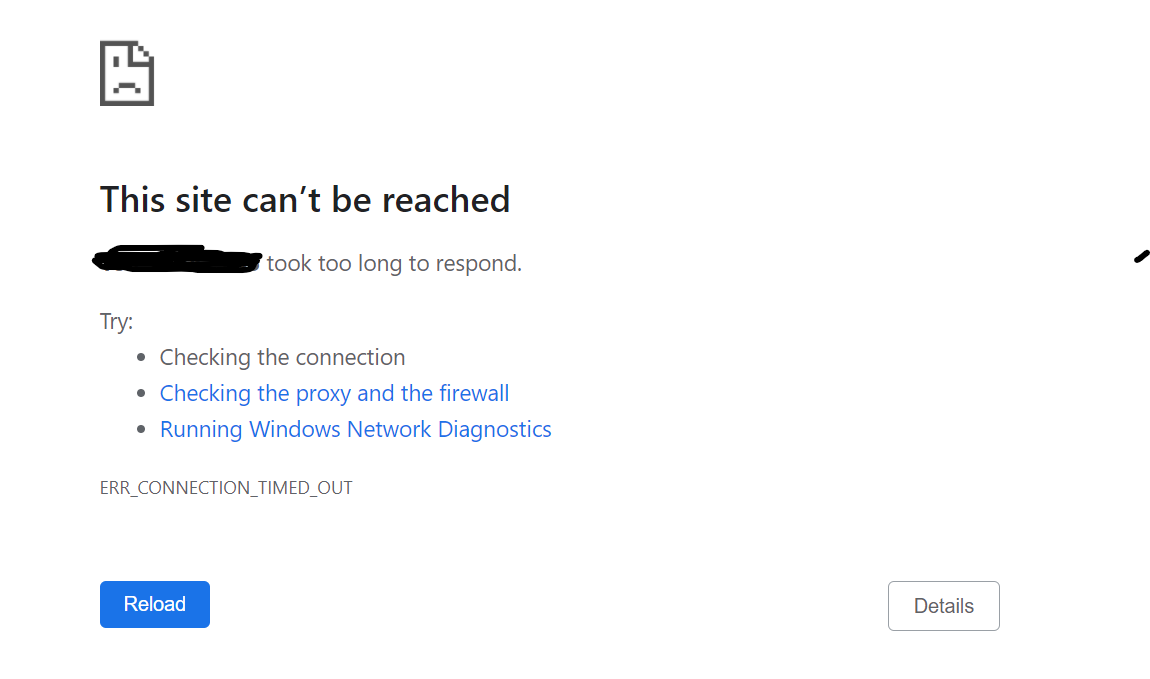This screenshot captures an error page displayed on a web browser. The background is predominantly white, featuring a simplistic design. On the far right edge, there's a thin vertical black line, likely part of the browser's user interface.

On the left side of the error page, there's a small icon of a piece of paper with one eye and a frowning face, capturing the user's attention. 

Below this icon, bold black text prominently reads: "This site can't be reached."

A slightly chaotic scribbled line is depicted underneath the phrase on the left side, signaling an area of disruption or emphasis.

To the right of the scribble, there is gray text that states: "took too long to respond."

Following this, another line begins with "Try...". Below this, several bullet points provide troubleshooting steps in blue, hyperlinked text:
- "Checking the connection"
- "Checking the proxy and the firewall"

An additional troubleshooting option is listed: "Running Windows Network Diagnostics," also in blue, hyperlink text.

At the very bottom of the page, there's an error code in all capitals: "ERR_CONNECTION_TIMED_OUT."

In the lower left-hand corner, a dark blue button with white text reads "RELOAD." On the right-hand side, another button with a light gray border and a white interior features the text "Details," with the letters 'R' and 'D' capitalized for emphasis.